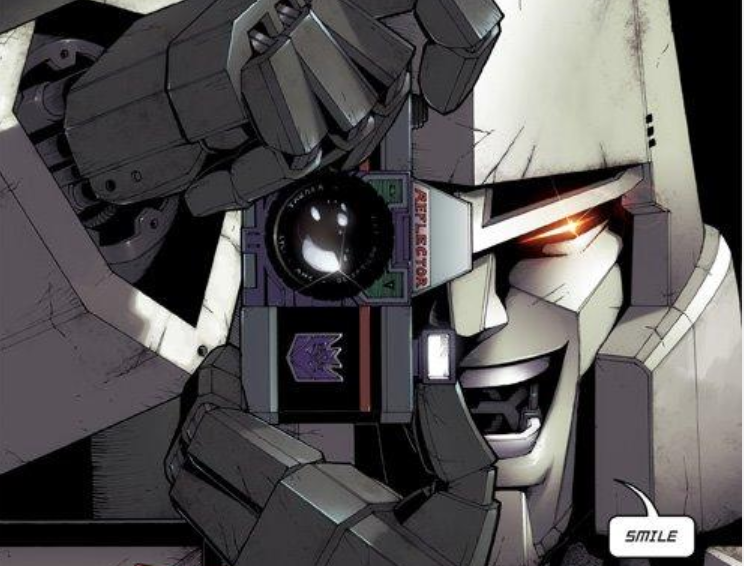This detailed and curated caption encompasses the shared and repeated elements across all voice descriptions, emphasizing the key details:

The image is a comic book-style illustration depicting a Transformer, likely from a Transformers comic book. The figure, clad in dark gray metal armor with a lighter gray sleeve, has glowing red eyes and appears to be smiling with an excited, almost sinister grin. The Transformer is holding a vintage-style DSLR camera with a flash bulb at the top and the Decepticon emblem on it. The camera itself is mostly silver with a distinctive black stripe on the side and a thin red stripe at the top, and it prominently features the word "Reflector" in red letters at the top. The camera is held vertically against one eye of the Transformer. Adding to the comic book feel, a speech bubble positioned at the bottom right of the image states "Smile," emphasizing the action. The overall color palette of the illustration is predominantly black, white, and gray, with the red elements on the camera and the transformer's eyes providing a stark contrast.